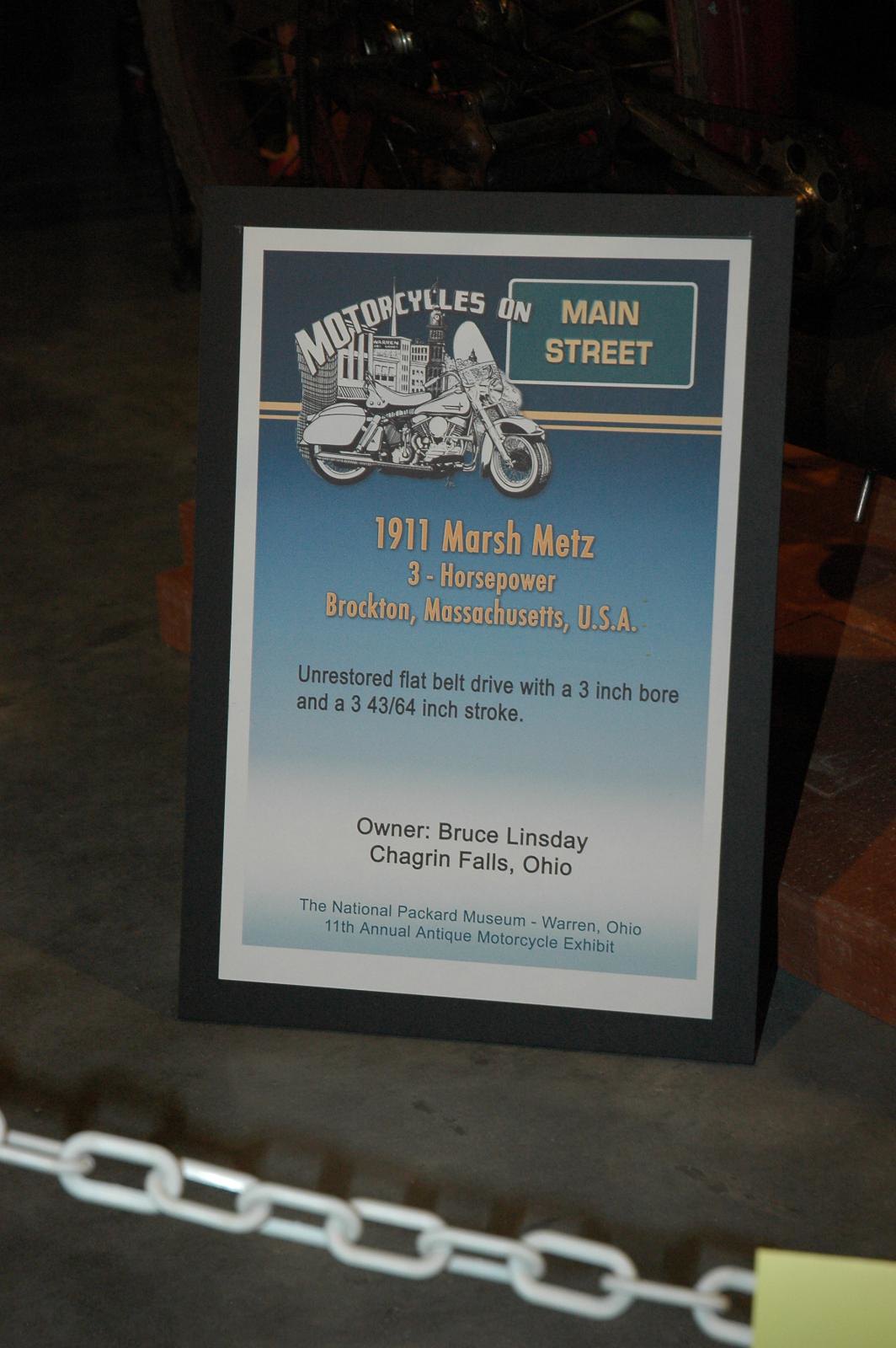This vertically aligned rectangular image features a street sign against a background that transitions from a blur at the bottom, revealing a white or gray chain link across dark gray ground that likely resembles cement. The central feature of the image is a framed sign with a black border, containing a white inner border. The sign's header reads "Motorcycles on Main Street" in white text, above a black-and-white motorcycle image positioned in front of buildings. Below this, in yellow text, it states "1911 Marsh Mets, 3 horsepower, Brockton, Massachusetts, USA." Further details, rendered in black text, describe the motorcycle as "unrestored flat belt drive with a 3-inch bore and a 3-43/64 inch stroke." At the sign's bottom, the owner is identified as "Bruce Lindsey, Chagrin Falls, Ohio," followed by information about the exhibit: "The National Packard Museum, Warren, Ohio, 11th Annual Antique Motorcycle Exhibit," presented in blue. The arrangement and detailed description suggest a convention or showcase setting, emphasizing the historical and technical specifics of the motorcycle on display.